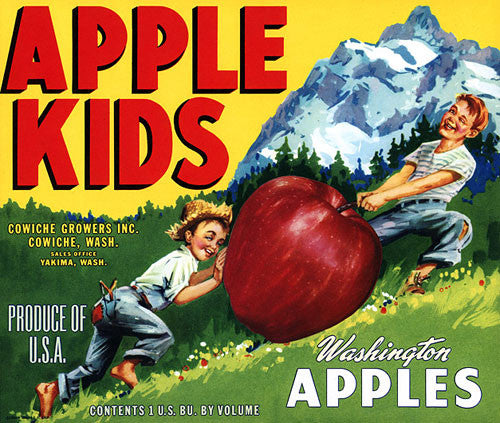This vibrant, artist-rendered advertisement for Washington Apples depicts an energetic outdoor scene set against a yellow sky and a prominent, snow-covered mountain in the background. In the foreground, two exuberant boys work together to move an oversized apple up a lush green hill. The boy at the bottom, who sports a straw hat, denim jeans, and a short-sleeved collared shirt, is barefoot and has a slingshot sticking out of his back pocket. He is pushing the apple up while gazing at the viewer with a wide smile. The boy at the top, also barefoot and dressed in denim jeans with a striped t-shirt, pulls the apple by its stem while looking at the viewer with a cheeky wink. Bold capital red letters in the top left of the image proclaim "Apple Kids," and smaller white letters in the bottom right announce "Washington Apples." The poster also includes text indicating "Produce of USA" on the bottom left, and beneath "Apple Kids," it reads "Cowich Growers Incorporated, Cowich, Washington," with a sales office located in Yakima, Washington.